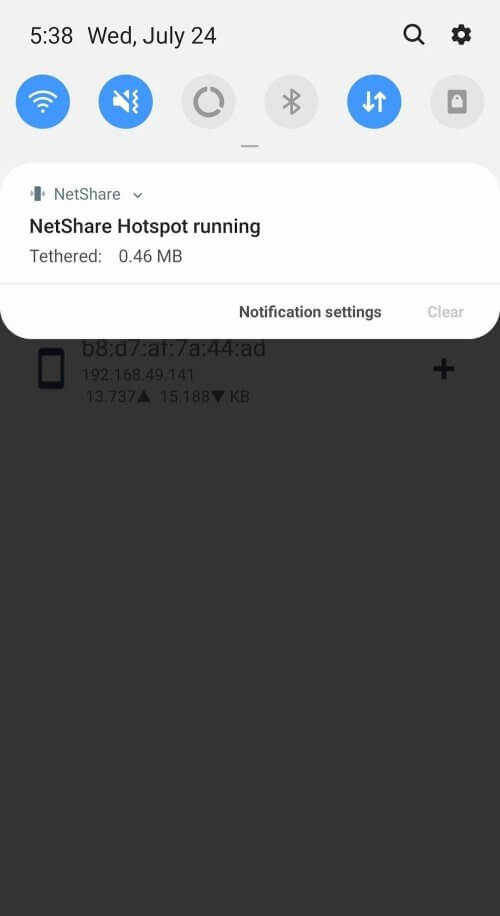In this detailed screenshot of an Android device's notification bar, we observe a variety of informational elements displayed. The timestamp at the top left corner reads "5:38 PM" on "Wednesday, July 24." On the top right, icons for a magnifying glass and a settings gear are visible. The status icons indicate that Wi-Fi is enabled and the ringer is turned off. Additional symbols include a circle, Bluetooth, an up-and-down arrow, a lock symbol, and a gray rectangle. 

Prominently, a notification from the "NetShare" application states, "NetShare hotspot running tethered 0.46 MB." At the bottom right of this notification, options for "Notification settings" and "Clear" are presented. Behind this notification, a grayed-out address "B8D7AF7A44AD" is partially visible alongside an IP address, "192.168.49.141." A small phone symbol is situated to the left of these alphanumeric codes.